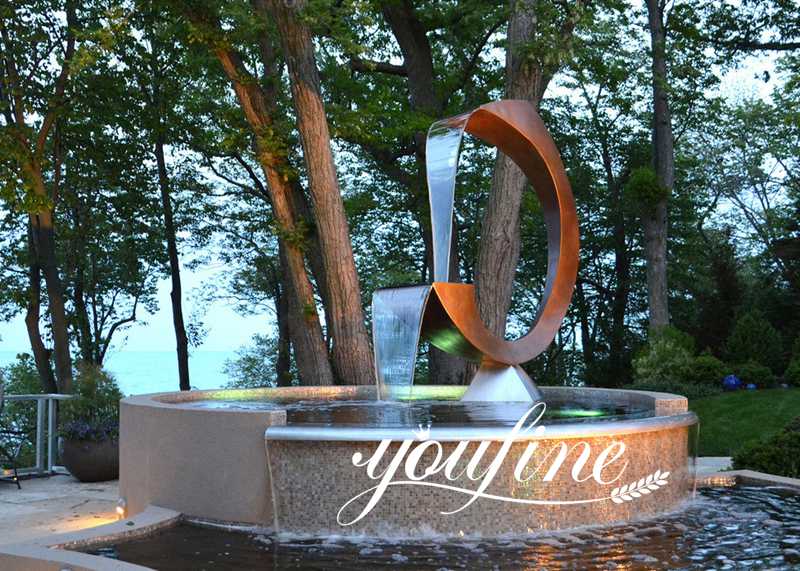The photo features an intricate bronze sculpture of a sea motif, doubling as a fountain. Water streams gracefully from the top, cascading over the sculpture’s sinuous curves before descending along the base, creating a secondary waterfall effect. The entire structure ultimately feeds into a larger fountain basin below, enhancing its dynamic flow. The word "Yuline" is inscribed in cursive at the front of the fountain, subtly blending with the sculpture’s light coloring due to the play of sunlight and shadow. The setting sun casts a warm glow, further highlighting the details of the artwork. Surrounding the fountain is a lightly wooded area, suggesting that this fountain is situated in a more natural, less urban environment, where trees and vegetation are allowed to grow freely.